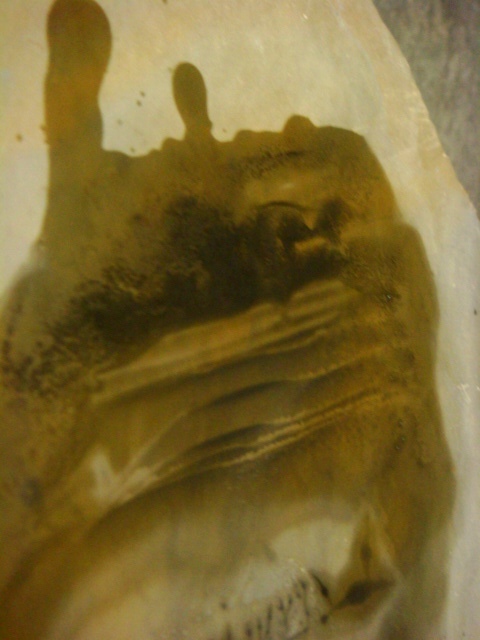The photograph features a blurred scene with no people, text, or date, set against a predominantly white background with hints of gray. The main focus is a central object, possibly a sheet of paper, resting on a grayish flooring. This object has a gold liquid, potentially molten gold or a mix of materials, splattered and dripping across it, creating intricate patterns of gold, black, and brown. Surrounding the central splatter are lighter off-white and cream hues, with some suggestions of a crystalline or rock-like structure. The image's indoor setting is dimly lit, with no signs of sunlight, and presents an enigmatic, almost abstract appearance.